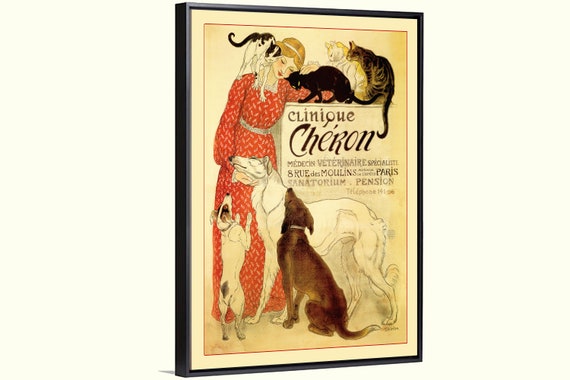The artwork depicted in this photograph is housed in a slender black frame with an off-white, slightly yellowed background. The image showcases a woman adorned in a floor-length, long-sleeved red dress with a silver waistband, indicative of the 1920s fashion. She has blonde, short hair styled with a headband, wearing bright red lipstick. The scene is bustling with pets: a black and white cat perches on her right shoulder, while she pets a black cat to her left. Beneath this group, a white dog is seen climbing up her leg. Just below these, a larger white dog and a slightly smaller brown dog sit on the ground, looking up at her. To the right, on a shelf labeled "Clinique Charon" in French, a collection of cats—ranging in colors from black to multicolored gray and striped—adds to the lively composition. The careful placement and interaction among the woman and her pets convey a warm, affectionate atmosphere.